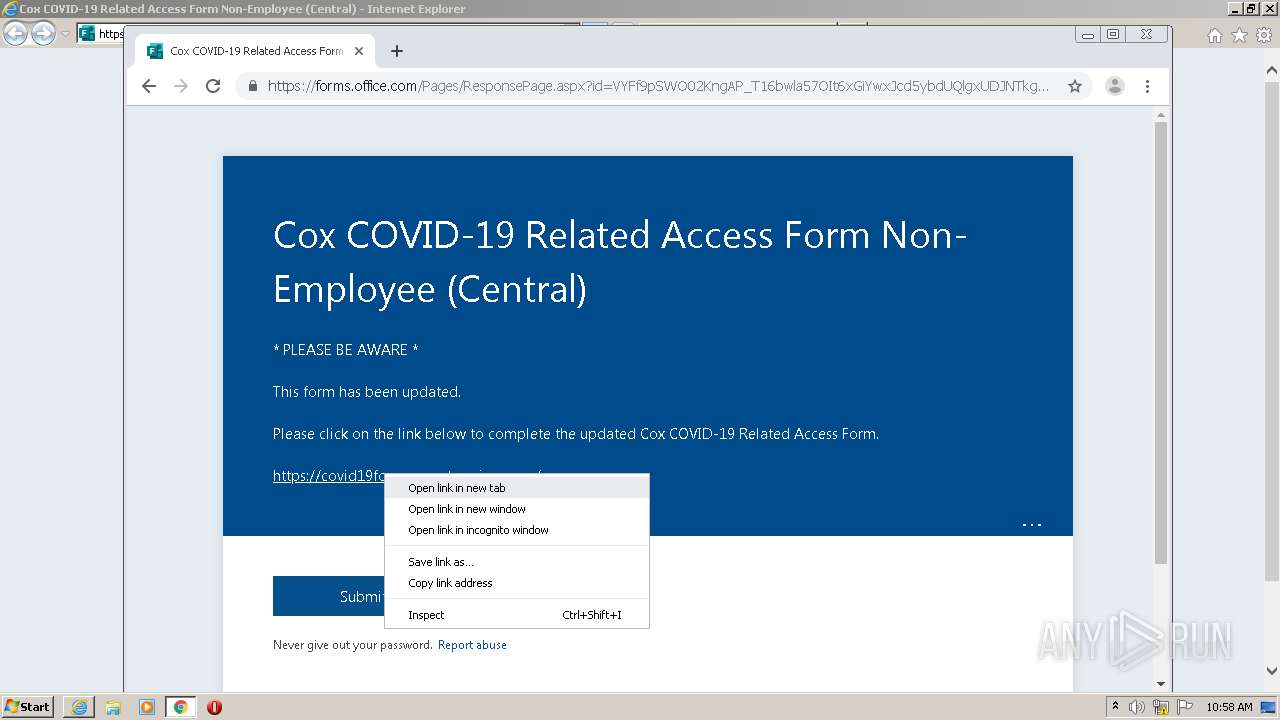The image depicts a screenshot of an Internet Explorer browser window where a user is interacting with a webpage on office.com, owned by Microsoft. The task involves completing a form related to Cox's COVID-19 access policies, specifically targeting non-employees. The form has been displayed within a large, nearly full-screen tab, but with slight cropping from the left and right margins and a small portion cut off at the top.

Dominating the webpage is a prominent blue box containing a notification: "Please be aware this form has been updated. Please click the link below to complete the updated Cox COVID-19 related access form." Beneath this notification, there is a clickable link and a submit button.

The user has right-clicked on the link, triggering a context menu to appear. This menu provides various options, such as "Open link in new tab," "Open in new window," "Open in incognito," "Save link as," "Copy link address," and "Inspect." The "Open link in new tab" option is highlighted, indicating the user's intention to open the form in a separate tab.